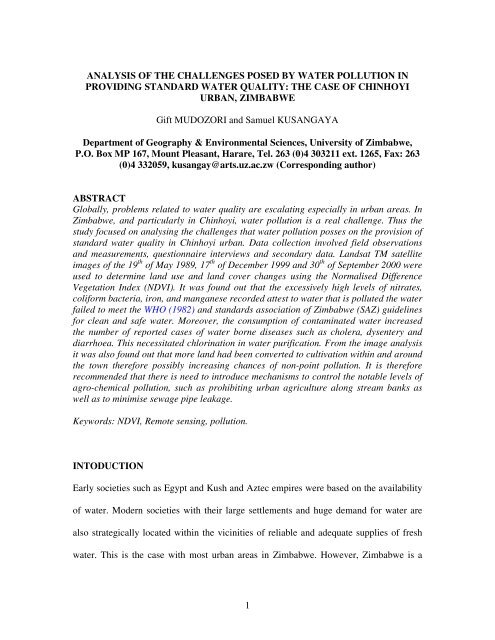This image shows a text document with small black text on a white background, likely from a scientific article or website. The title reads, "Analysis of the Challenges Posed by Water Pollution in Providing Standard Water Quality: The Case of Chinhoyi, Urban Zimbabwe," authored by Gift Muto, Zori, and Samuel Kusangaya from the Department of Geography and Environmental Sciences at the University of Zimbabwe. Their contact details are also listed. The abstract outlines the global escalation of water quality issues, particularly in urban areas of Zimbabwe like Chinhoyi, emphasizing challenges with nitrates, coliform bacteria, iron, and manganese levels in water, which failed to meet WHO 1982 and Standards Association of Zimbabwe guidelines. The consumption of contaminated water has increased waterborne diseases, necessitating water purification efforts. The study used Landsat TM satellite images to analyze land use changes, revealing increased agricultural activity near the town, contributing to nonpoint pollution. The introduction notes that, historically, civilizations like Egypt, Kush, and the Aztec empires thrived on water availability, and modern urban areas in Zimbabwe similarly depend on reliable freshwater sources, noting Zimbabwe's ongoing struggle with water quality issues. The page is identified as part of a longer document, indicated by a "1" at the bottom.